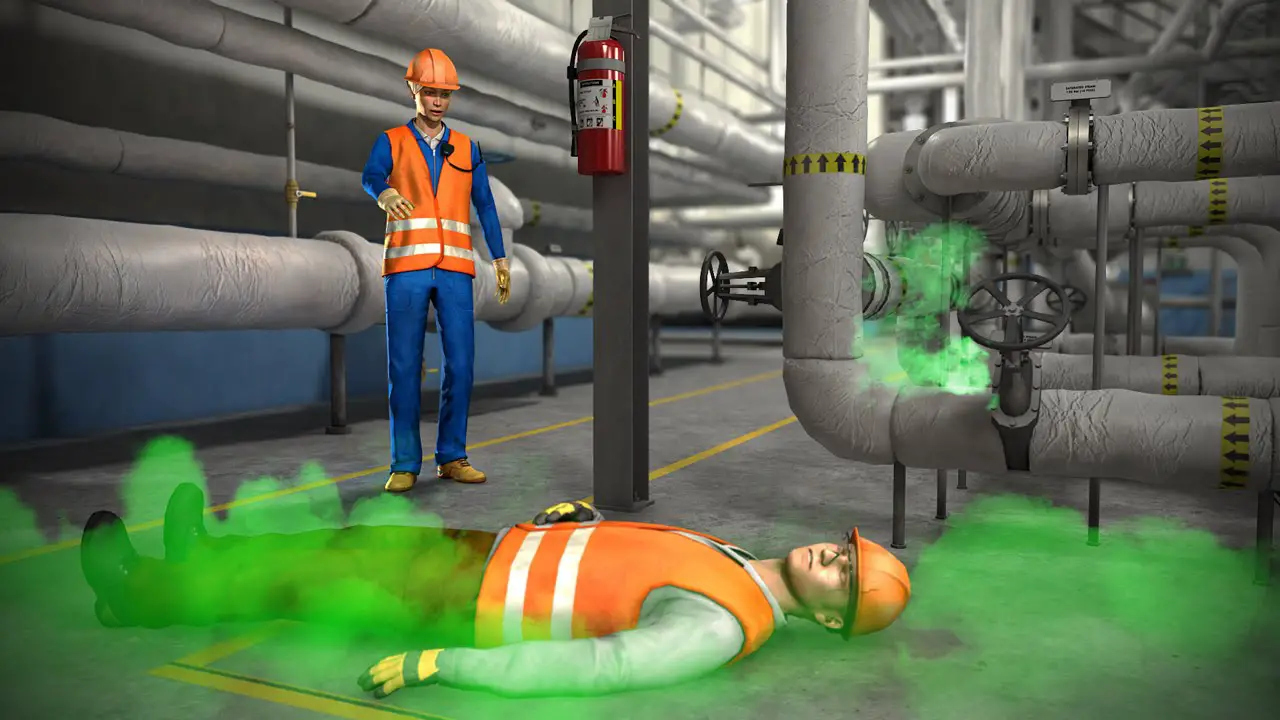In this highly detailed, computer-generated image reminiscent of a 3D video game or animated scene, we find ourselves in a bustling factory setting filled with intricate piping systems. Large, gray pipes dominate the backdrop, some adorned with yellow and black arrows pointing in various directions, hinting at the complex gas or liquid flows within. The environment evokes an intense industrial ambiance, suggested by the multitude of interconnected pipes and mechanical elements.

At the forefront of this scene, two workers in bright safety gear command attention. Both men don orange vests with white stripes, orange safety helmets, and yellow gloves, marking them as crew members engaged in potentially hazardous work. One of the workers, wearing black pants, lies prone on the ground, his right hand clutching his stomach amidst an ominous cloud of green gas escaping from the nearby pipes. His position and the green fumes suggest either a severe injury or exposure to a toxic substance.

Standing near him is another worker, distinguished by his blue trousers and yellow shoes. This gentleman, who appears alarmed and concerned, is looking intently at his fallen colleague. His tense posture underscores the gravity of the situation. Positioned between them is a black pole adorned with a conspicuously attached red fire extinguisher, alluding to the safety protocols in place despite the apparent accident.

Overall, the image masterfully captures a moment of crisis within a constrained industrial environment, blending vibrant safety colors with the muted grays of the factory apparatus, and emphasizing the urgency of the scene with the escaping green gas and the workers’ heightened states of alert.